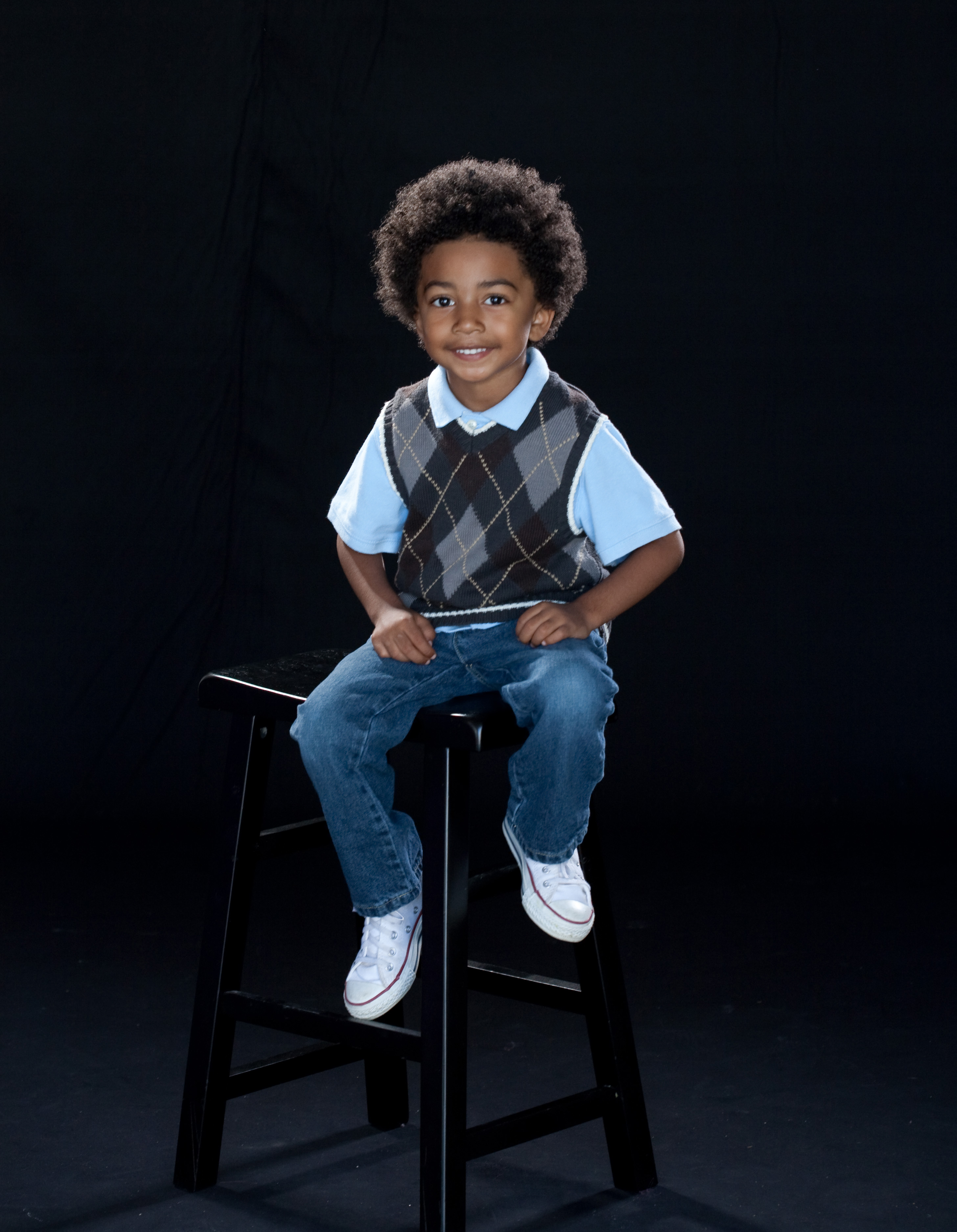The photograph captures a small child seated on a tall square-shaped bar stool, which is nearly as tall as the child itself. The child has short to medium-length curly black hair and is seated with their hands resting on their upper legs. They are facing forward, smiling broadly to reveal their front upper row teeth, and gazing directly at the camera with their black eyes. The young child is dressed in a short-sleeved light blue polo t-shirt, fully buttoned, and layered with an argyle patterned sweater vest featuring black, yellow, and gray diamonds. Complementing this outfit, they wear blue jeans and white shoes with distinctive brown bands between the soles and the sides. The scene is set against a seamless black backdrop, making it difficult to distinguish where the floor ends and the wall begins, although the floor appears to be a dark gray color. The stool, which has four legs, blends into this dark environment, centering the child perfectly within the composition.